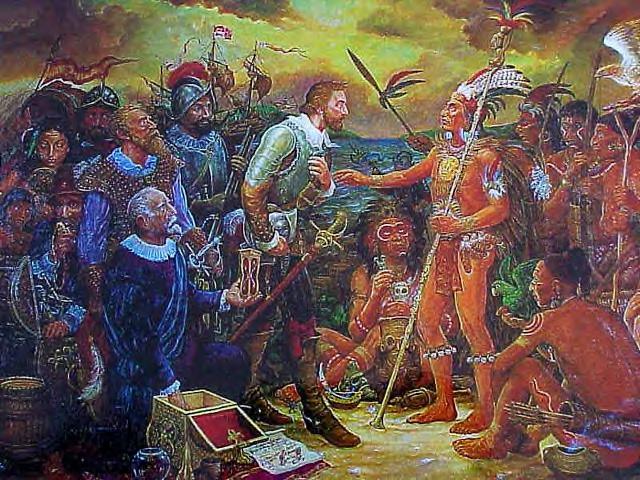The painting vividly depicts a historical encounter between Spanish conquistadors and indigenous people of the Americas. The scene unfolds on a colorful beach with large sailing ships anchored in the background. The Spanish, identifiable by their distinctive helmets reminiscent of the Spanish Armada, are presenting treasures and gifts from chests to the native people. Among the Spanish group, a woman is present, and a flag, albeit indistinct, flutters on one of the ships. The indigenous people, some sitting and others standing, are adorned in brightly colored headdresses, gold jewelry, face paint, and loincloths. The lead native figure, possibly a chief, stands prominently, extending his arm towards the Spaniards. He wears a headdress colored red, green, and white, reminiscent of the Mexican flag, and holds a staff adorned with feathers and a perched bird. Other natives are equipped with bows, arrows, and additional staffs with feathers. The interaction is rich in cultural detail, capturing a moment fraught with tension, curiosity, and significance. The vivid colors and intricate details draw the viewer into the complex tapestry of this historical meeting.